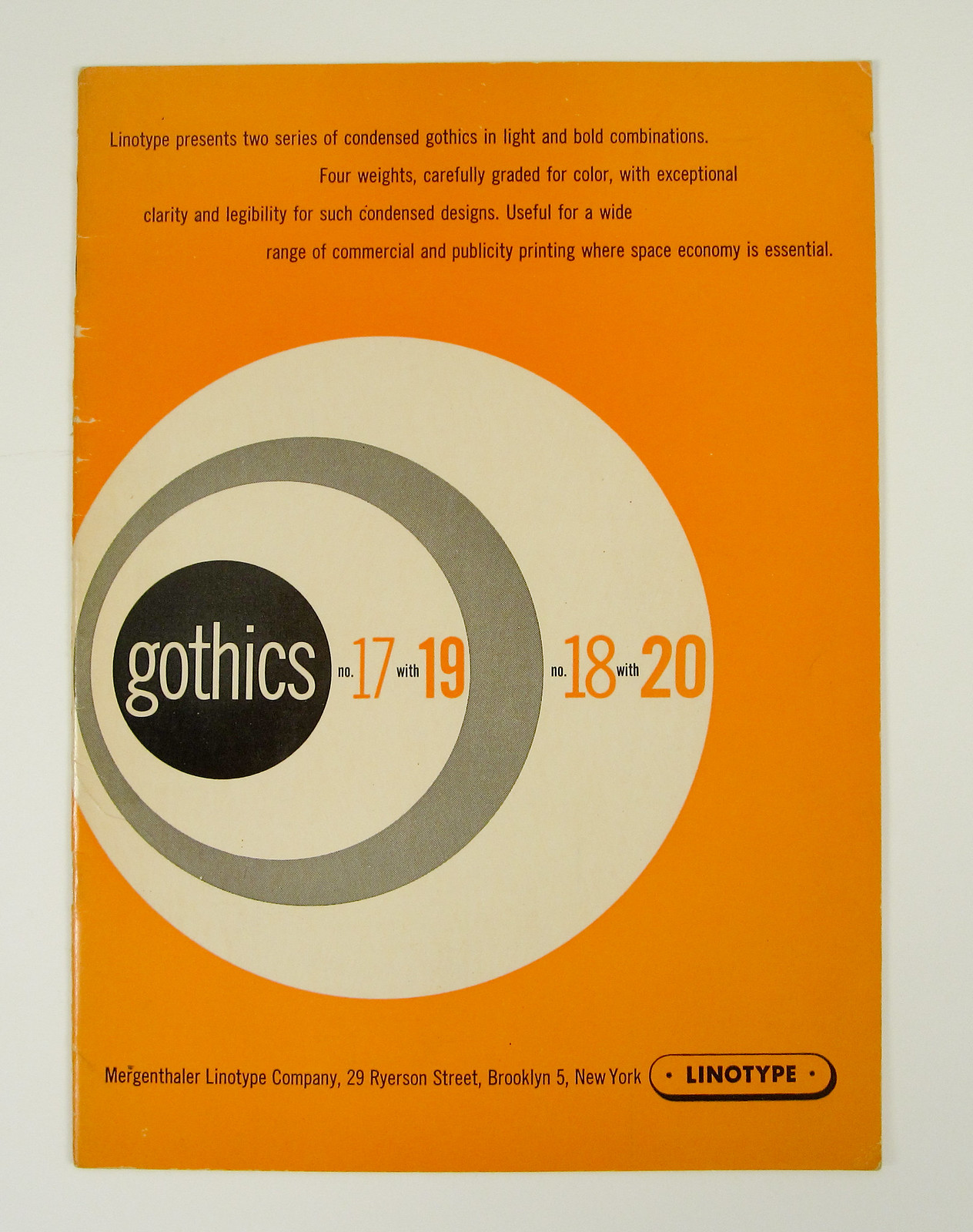This color image showcases an old advertisement for typesetting, dominated by a palette of orange, white, black, off-white, and gray. Serving as the cover for a booklet or brochure, it prominently features "Linotype presents two series of condensed gothics in light and bold combinations" at the top. It declares the availability of four carefully graded weights designed for optimal color, clarity, and legibility despite their condensed format. The ad highlights their utility in various commercial and publicity printing scenarios where space efficiency is crucial. 

Central to the design, four concentric circles vary in color: black, white, gray, and white again, all situated slightly to the left. Running through these circles are the names of the gothic typefaces: gothics 17, 19, 18, and 20. At the bottom, the ad lists the Mergenthaler Linotype Company, located at 29 Ryerson Street, Brooklyn 5, New York, with "Linotype" prominently displayed in bold letters in the bottom-right corner. The overall design underscores traditional printing aesthetics and meticulous attention to typographic detail.